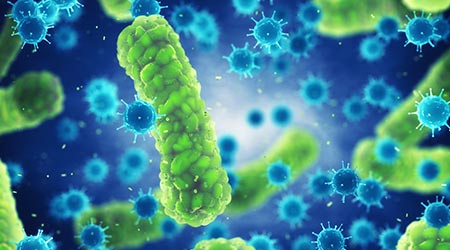The image is a computer-generated depiction often seen in medical articles as a stock photo. It portrays a microscopic view of what appears to be an immune system response to pathogens. The background is a dark blue abyss with a bright spot in the middle, suggesting a light source. The scene is populated by tens of spiky blue orbs, each resembling a white blood cell, attacking lime green structures. These green objects have a pill-like shape, with nodules along their forms, resembling caterpillars. The color palette includes shades of green, blue, white, and some black, creating a stark contrast. The image lacks any text or context, leaving its interpretation open, but it effectively conveys a microscopic battle between immune cells and pathogens.